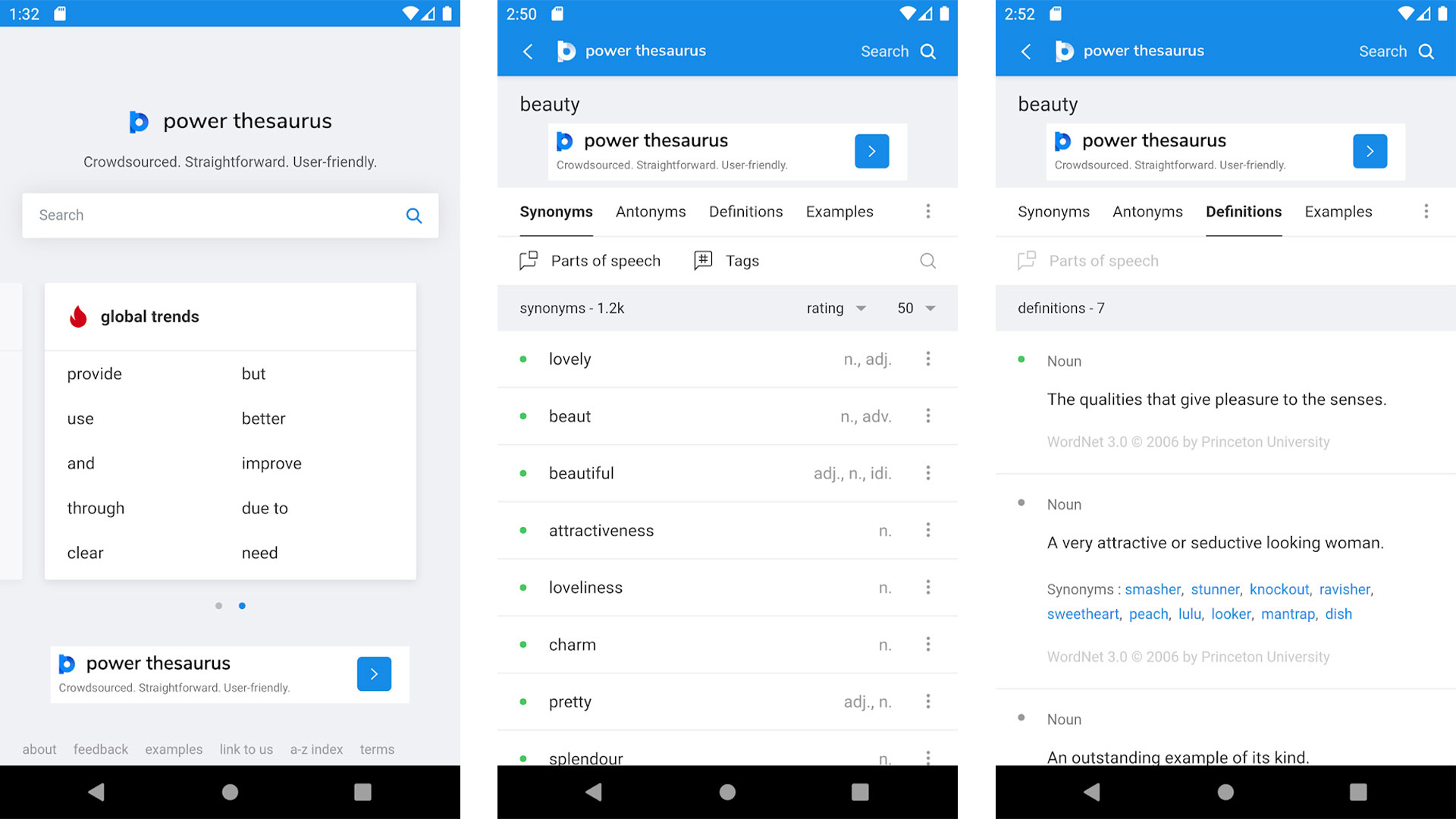The image consists of three side-by-side panels, each resembling the screen of a mobile app. Here's a detailed description of each panel:

**Left Panel:**

- **Top Bar:** A thin blue banner occupies the top. The left side displays the time "1:32," while the right side features icons for a SIM card, battery, Wi-Fi signal, and cell signal.
- **Main Content Area:** 
  - The background is a light blue or light gray.
  - A small letter "P" appears followed by "power thesaurus" in all lowercase letters.
  - Below "power thesaurus," the text "crowdsourced, straightforward, user-friendly" is displayed.
  - A search bar with a blue magnifying glass icon is present.
  - Below the search bar is a white square displaying a red flame icon with the label "global trends."
  - A list of trending words is shown, including "provide," "use," "through," "clear," "better," "approved," "due," and "meet."
  - The bottom of the panel contains a blue banner with the text "power thesaurus."

**Middle Panel:**

- **Top Bar:** A thicker blue banner similar to the left panel, with the time "2:50" and the same icons on the right.
- **Main Content Area:**
  - The header reads "power thesaurus," alongside a left-facing arrow on the left side.
  - The word "beauty" is highlighted in a gray background.
  - Beneath it, a blue banner reads "power thesaurus, crowdsourced, straightforward, user-friendly" with a blue square and right-facing arrow icon.
  - Following the blue banner, the words "synonyms, antonyms, definitions" are listed, with "synonyms" in bold.
  - A list of synonyms for "beauty" follows: "lovely," "beautiful," "attractiveness," "loveliness," "charm," "pretty," and "splendor."

**Right Panel:**

- **Top Bar:** A blue banner identical to the previous panels, along with the same time and icons.
- **Main Content Area:**
  - The word "beauty" is once again the focal point.
  - Below it, "power thesaurus" is mentioned.
  - The terms "synonyms, antonyms, definitions, examples" are listed, with "definitions" in bold.
  - A detailed definition of "beauty" is provided:
    - **Noun:** The qualities that give pleasure to the senses.
    - **Noun:** A very attractive and respectable-looking woman.
    - **Noun:** An authentic example of its kind.

This narrative provides a coherent and meticulous description of the three panels, encapsulating the interface elements and textual content comprehensively.